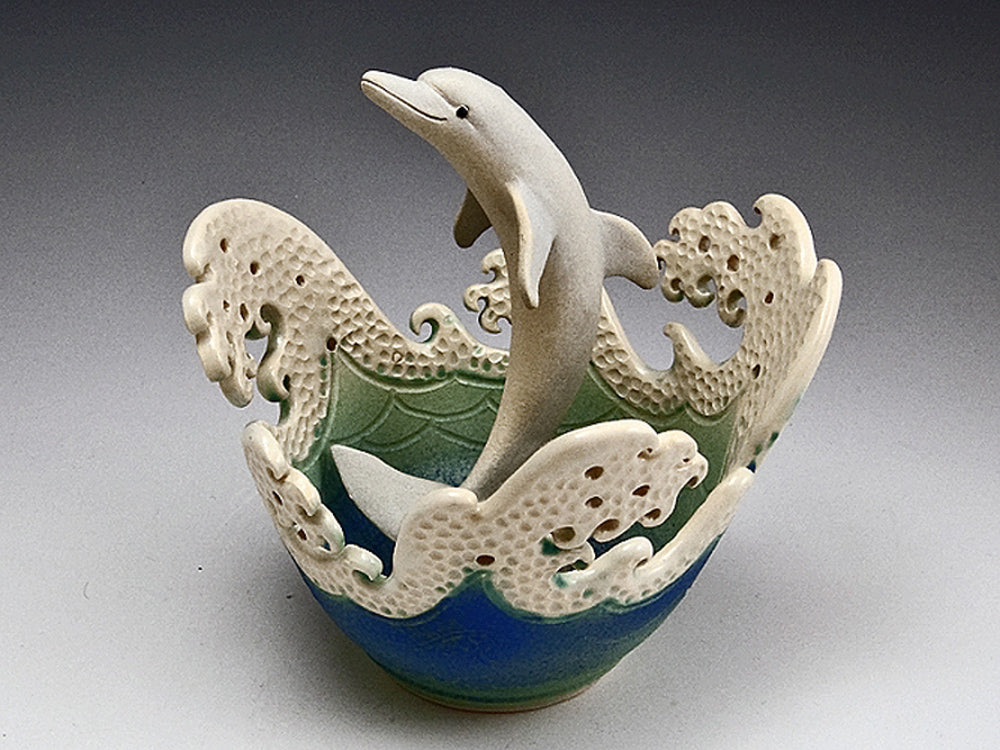This is a detailed photograph of a unique ceramic bowl designed to resemble ocean waves with a playful dolphin centerpiece. The bowl features a gradient from deep blue at the base, transitioning into green, capturing the essence of ocean depths. The exterior of the bowl portrays frothy white waves with a textured, hole-filled surface, rising intricately around the edges. These ceramic waves continue inside the bowl, where the greenish hue deepens the aquatic theme.

Soaring out of the center is a gray dolphin, complete with a cheerful expression and a black dot for its eye, adding charm to the piece. The dolphin's detailed flippers and tail are made of the same ceramic material. The bowl rests on a gradient background that transitions from black at the top to white at the bottom, enhancing its visual appeal. This bowl could serve as an enchanting candy dish or a decorative item likely to delight both children and adults alike.